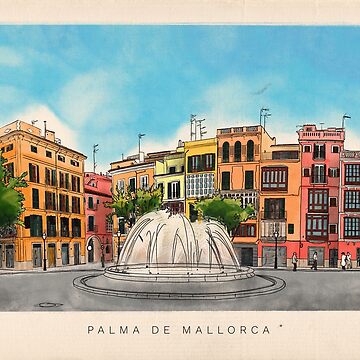This detailed illustration, reminiscent of a postcard or tourist pamphlet, depicts a vibrant scene from Palma de Mallorca. In the foreground, a large circular fountain gushes water, set against a gray pavement. To the left and center of the image, colorful buildings rise with facades painted in shades of orange, pink, and yellow. These structures, likely serving as storefronts, apartments, hotels, or hostels, are four to five stories tall and feature numerous antennas on their rooftops. Between the fountain and the buildings, there are three lush green trees and several lampposts lining the sidewalk. A few pedestrians stroll along the right side of the scene. Overhead, a blue sky dotted with fluffy white clouds provides a tranquil backdrop to this bustling downtown area, which is drawn in a bright, cartoonish style that could also suggest its use as an album cover.